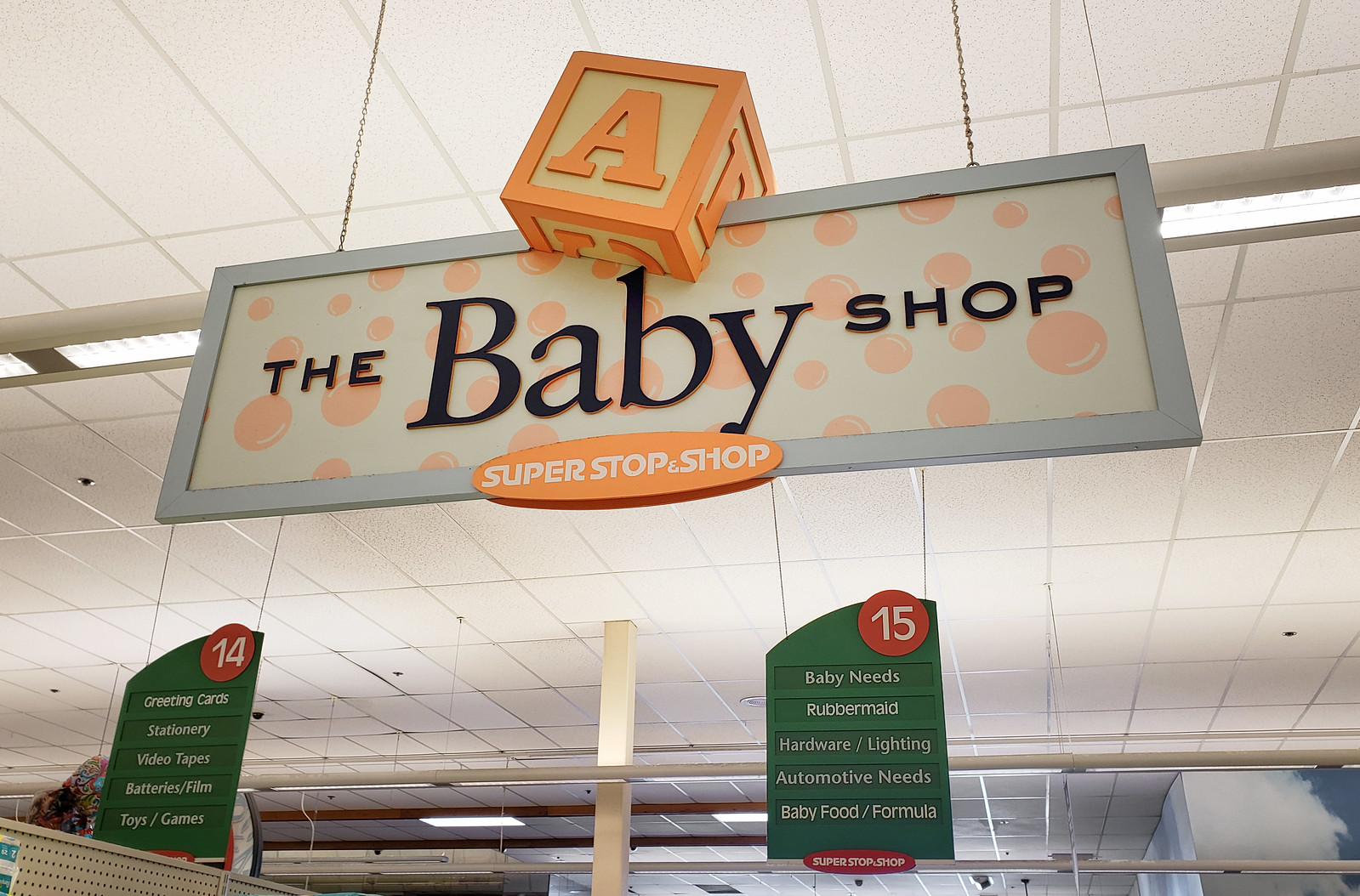In this color photograph, the viewer is presented with a snapshot of the interior of a store. The image is slightly wider than it is tall, with the focus directed upward towards the store's ceiling. Prominently featured is a sign suspended from the ceiling, demarcating the section dedicated to baby products. The sign is rectangular, with the words "The Baby Store Shop" clearly visible. Below this main sign, an oval-shaped piece hangs, displaying "Super Stop" in white letters, making it a notable feature within the store's signage.

Adorning the top of the sign, there is a motive of a baby block, adding to the thematic representation of the section. The store's interior roofing is white, providing a bright backdrop that contrasts with the sign. In the photograph's lower left section, the number "14" is visible, indicating the aisle number, though the actual contents of that aisle are not clearly readable. On the right side, aisle number "15" is marked with a green hanging sign from the ceiling, though its details are also obscured. This image captures the organized layout typically seen in stores, highlighting the baby product section within the broader store environment.